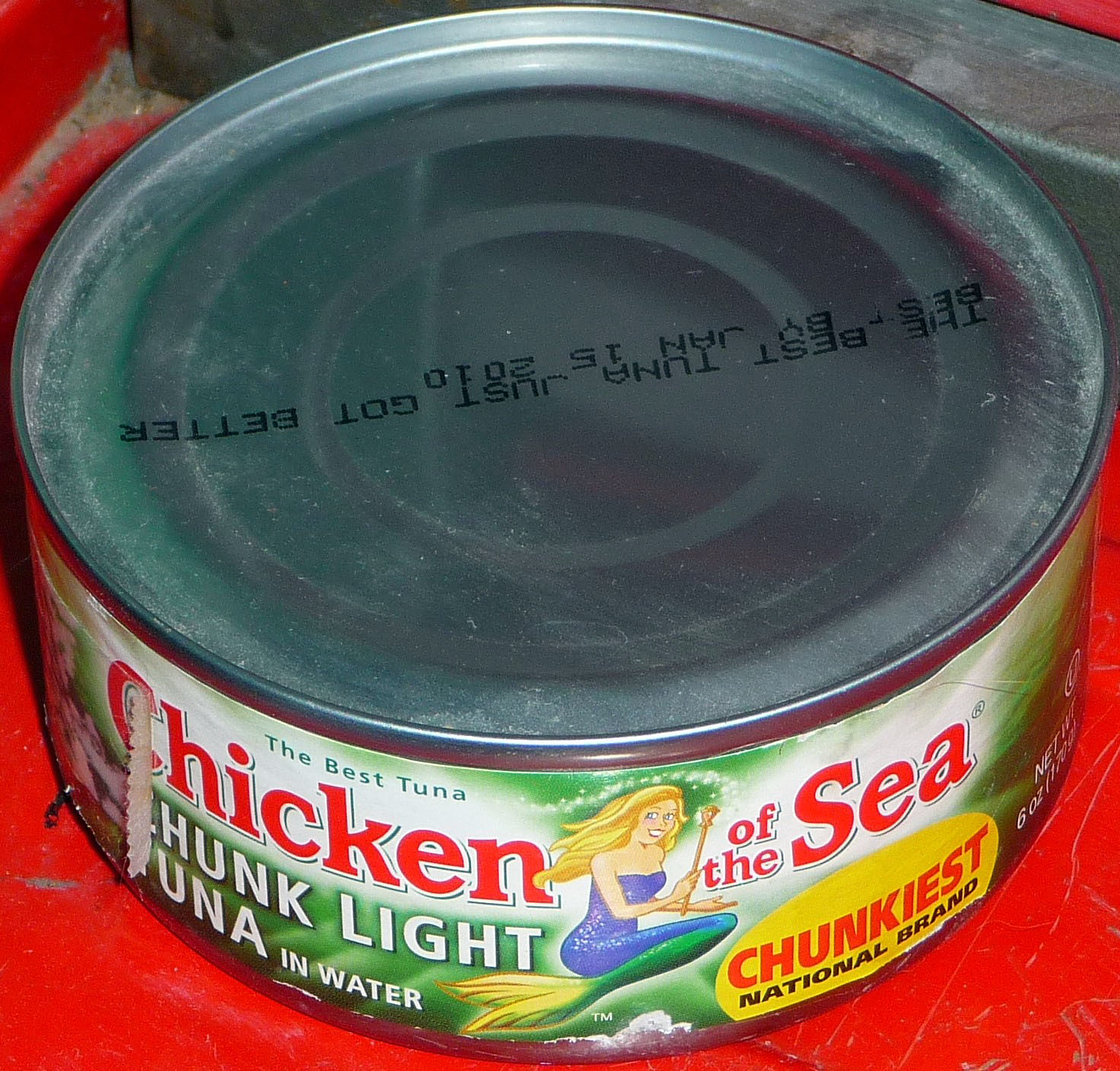This angled overhead photograph captures a can of Chicken of the Sea tuna prominently situated within a red-painted metal container or drawer. The top of the can, coated with a layer of dust and dirt, indicates that it has been stored for an extended period. The label predominantly features shades of green, accented with red and white text, announcing "The Best Tuna Just Got Better" and "Chunk Light Tuna in Water." Additionally, it touts the slogan "Chunkiest National Brand." Notably, the can's lid includes a "Best By" date of January 15, 2010. Adorning the label is an illustration of a blonde Caucasian mermaid, who holds a wand emitting bubbles and light. Her form transitions from a human torso to a fishtail below the armpits, with the tail shading from blue to green around the knee area. This image poignantly captures a well-worn item amidst a scene of neglect.